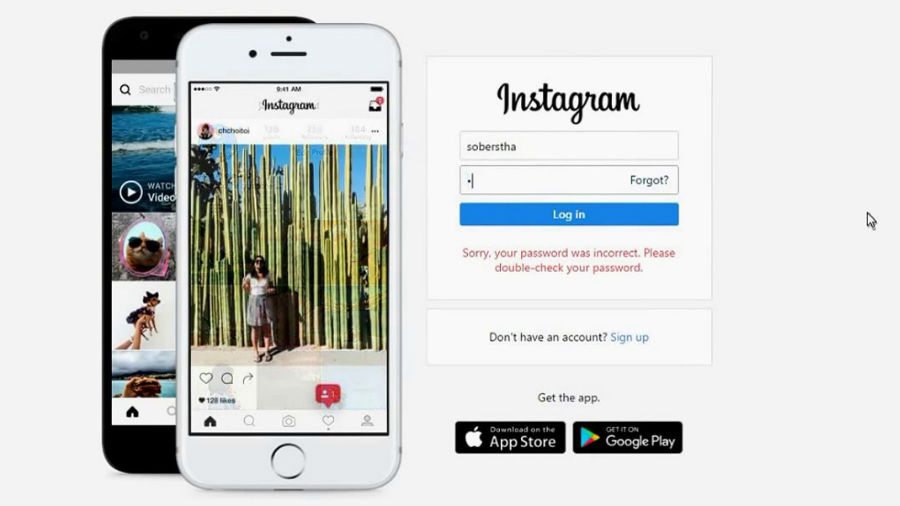The advertisement image for Instagram features two older model iPhones prominently positioned on the left 40% of the frame. A white iPhone, partially obscuring a black iPhone behind it, displays the Instagram app interface. Both iPhones have physical home buttons, indicating their older models.

To the right, occupying the remaining 60% of the image, is a login box for Instagram. The login interface includes fields for username and password, with a blue "Log In" button displaying white text just below. An error message underneath reads, "Sorry, your password was incorrect. Please double-check your password."

Beneath the login box is a smaller box prompting users with "Don't have an account?" followed by a hyperlink encouraging new users to "Sign up."

Further down, two icons invite users to download the app. The left icon shows the Apple App Store logo with "Download on the App Store," and the right icon displays the Google Play Store logo with "Get it on Google Play."

The overall background is a neutral gray, with the leftmost 10% and rightmost 20% of the image margins being blank, devoid of any text or additional imagery. This layout appears to simulate the typical Instagram login screen.